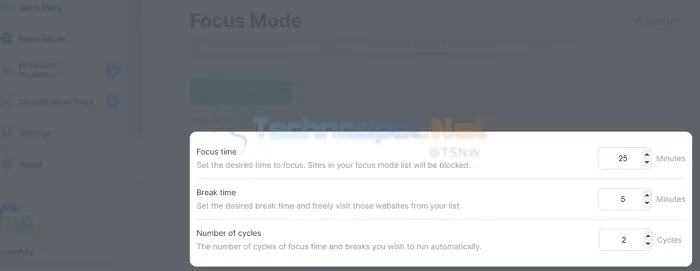The screenshot displays a somewhat unreadable interface because it's obscured by a translucent overlay with a grey-blue hue, creating a very dark and blurry visual. 

At the center of the obscured screen, "Focus Mode" is prominently displayed in large, bold black text. In the lower right corner of the screenshot, there is a large white pop-up panel with three main sections: "Focus Time," "Break Time," and "Number of Cycles."

Under "Focus Time," it instructs to "set the desired time to focus" and mentions that sites in your focus mode list will be blocked. The current setting shows 25 minutes, which can be adjusted using up and down arrows to the right of the input field.

The "Break Time" section allows you to "set the desired break time" during which you can freely visit websites from your list. The break duration is set to 5 minutes, with similar adjustment arrows available beside the input field.

Finally, "Number of Cycles" refers to the number of focus and break intervals you wish to automate, set to 2 cycles by default, with corresponding up and down arrows for adjustments.

This feature might be particularly useful for individuals seeking help to manage their self-discipline and stay productive by defining and enforcing periods for focused work and breaks.